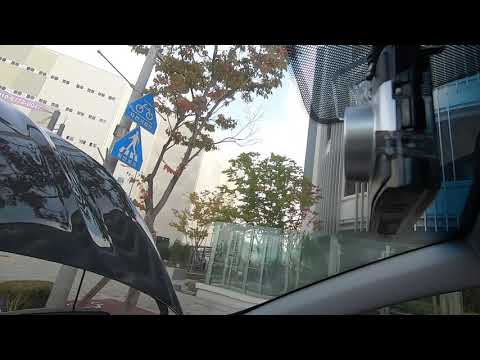The image depicts a cityscape viewed from inside a vehicle, specifically from behind the windshield and partially seeing the open hood, which is black and shiny. The car's view is obstructed on the right side by a metal or plastic object, possibly a GPS or dash cam. In the foreground, there's a rearview mirror and part of the windshield visible. Directly ahead, a white or gray telephone pole stands, adorned with two triangular signs: one depicting a cyclist and the other showing a pedestrian on a crosswalk. The scene also includes a variety of urban elements on the right side, such as the sidewalk, a mix of buildings, and a tree with orange and green leaves. In the background, larger buildings loom, with one having three rows of small windows. A stretch of fencing and additional thin trees with yellow or green leaves can be seen further behind. The sky is predominantly white with only a faint touch of blue.